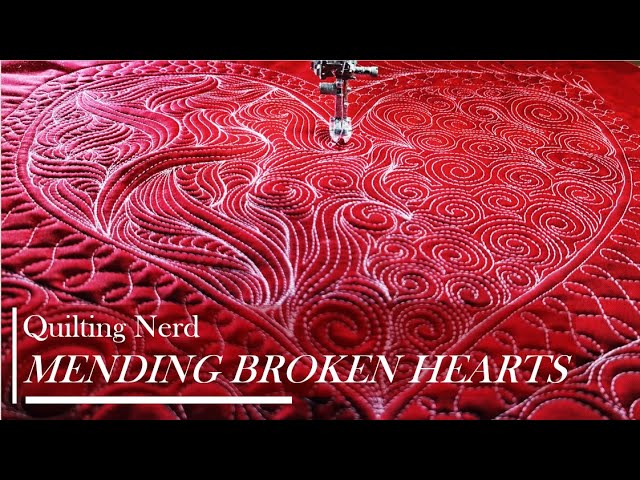The image depicts a beautifully detailed quilting project showcased on a dark background. Central to the image is the foot of a sewing machine, intricately stitching a large, vibrant red heart onto the fabric. The heart, quilted with elegant swirls and curlicues, is crafted with meticulous white thread. The left side of the heart features vine-like, twisty stitches, while the right side showcases a series of curlicues, creating a dynamic and non-uniform pattern. This intricate heart is framed by a border of figure eights or infinity symbols. The quilt fabric has a satin sheen, giving the red a blood-like vibrancy. Towards the bottom right corner, the image bears the text "Quilting Nerd, Mending Broken Hearts," emphasizing the theme of creativity and emotional repair through quilting. This stunning visual exemplifies the beauty and potential of machine quilting, with the subtle puckering of the stitches adding depth and texture to the design.